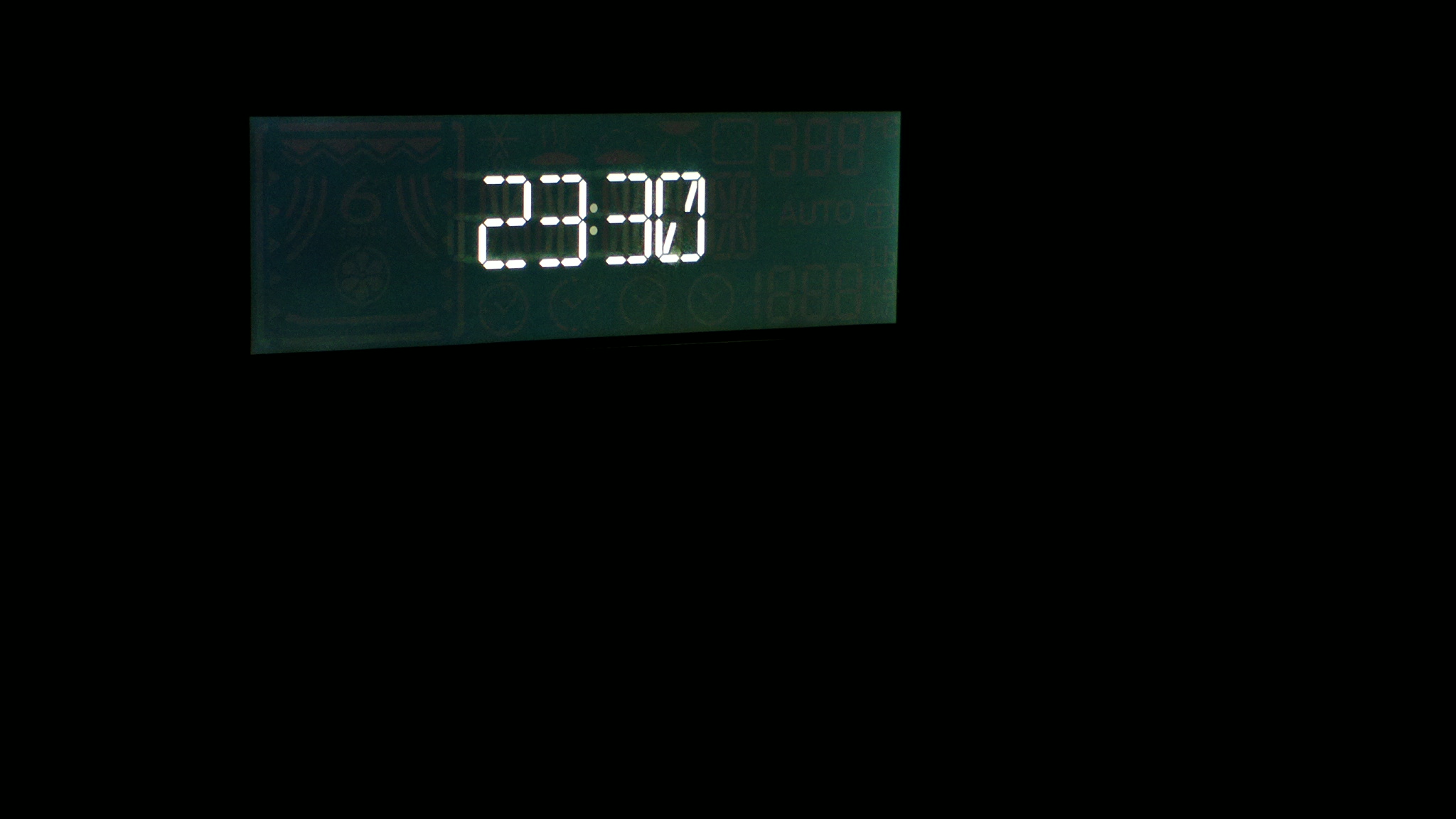The image presented is a rectangular field, wider than it is tall, dominated by a solid black backdrop. In the top left corner of this dark expanse, a rectangular LED screen, oriented wider than it is tall, captures attention. The screen prominently displays white illuminated numbers reading "23:30," suggesting the time is 11:30 PM. The LED digits exhibit a slight greenish hue, more pronounced on the right side of the screen. Additionally, a subtle ghosting effect is visible around the numbers, potentially indicating a reflection or minor motion blur when the photograph was taken. The rest of the image remains a uniform, unbroken black.